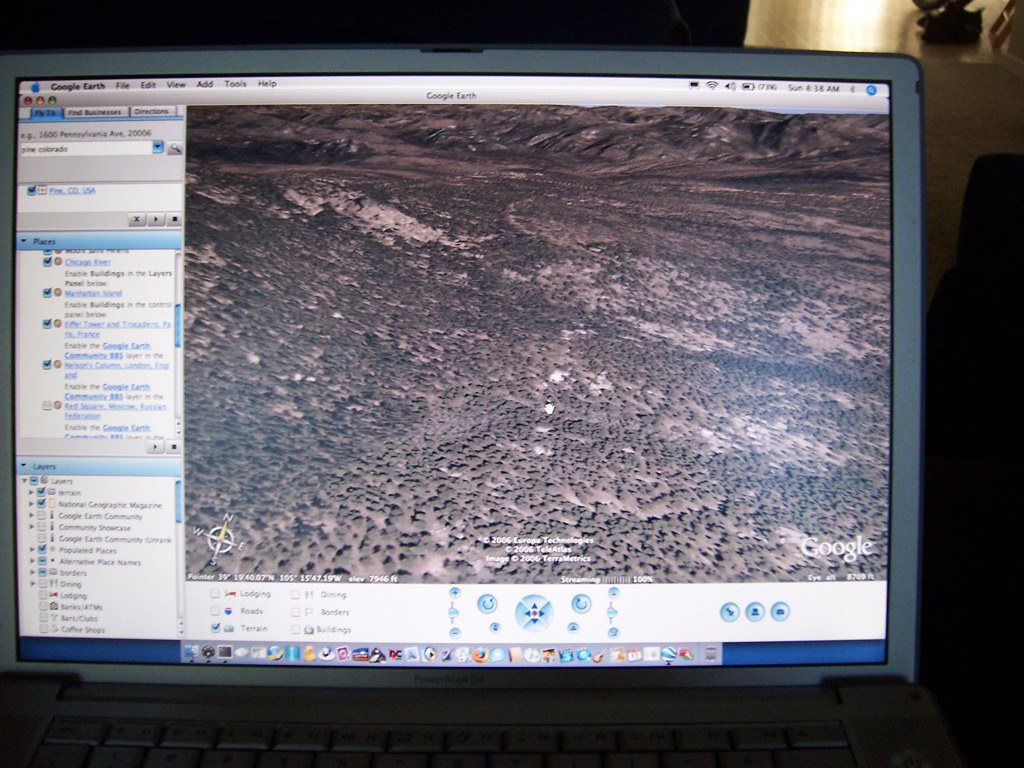The image depicts a laptop, partially showing its keyboard and fully displaying its screen. The keyboard is only visible up to about half of its layout. The screen prominently features an open Google Earth application, showcasing a detailed topographic map. The terrain displayed on the screen consists of extensive hills and small mountains, characterized by shades of brown, suggesting a dry or arid region. Sparse patches of grass can be identified, though they lack a vibrant green color. No bodies of water are present within this view. Additionally, a compass icon is visible at the bottom of the screen, indicating directional orientation.